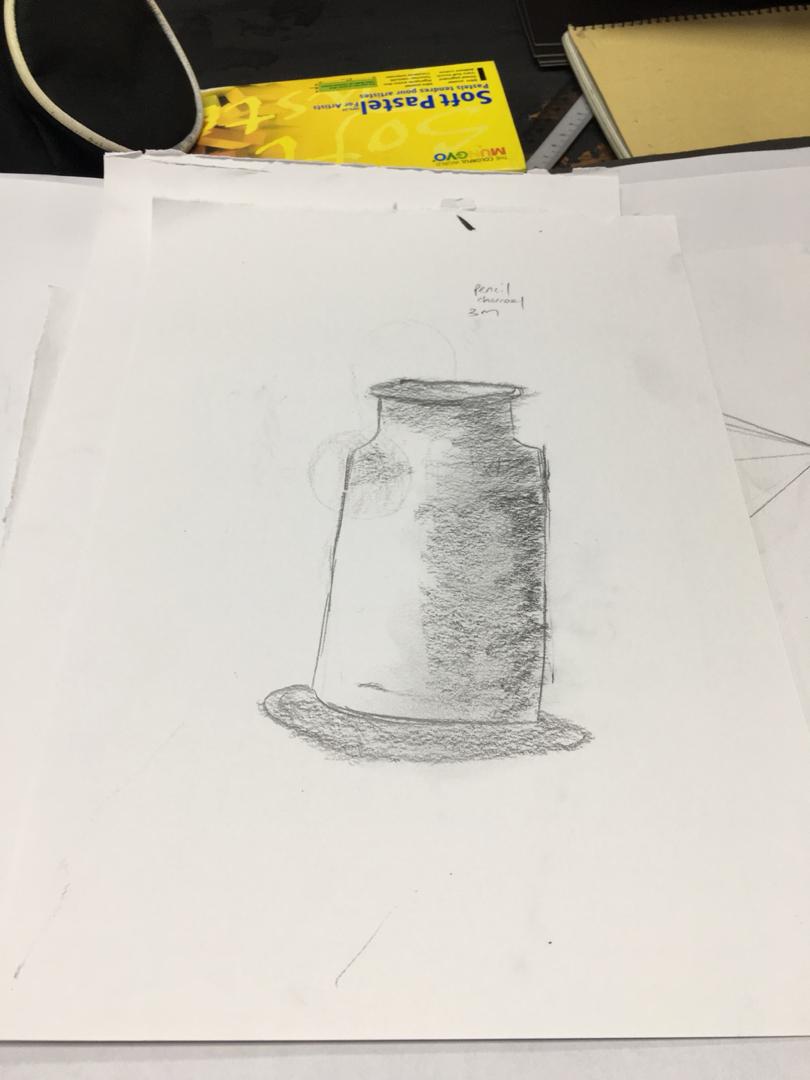The color photograph captures a detailed charcoal drawing on a white sheet of paper. The drawing depicts what seems to be a milk jug or a small square vase with a rounded top, complete with intricate shadowing that emphasizes the darker, right-hand side and a drop shadow beneath it. At the upper right corner of the paper, the words "pencil, charcoal, 3M" are inscribed, though some text may be illegible. The setting includes a white desk or table covered with various items: a clear triangular implement, a small steel rule, and an additional notebook with a brown spiraled cover. An electrical cable or power cord extends from the top left corner. Prominently in the background is an upside-down yellow box labeled "soft pastel" in blue letters, suggesting it contains art supplies. The overall scene is meticulously arranged, with light coming from the left, casting distinct shadows and adding depth to the sketch.